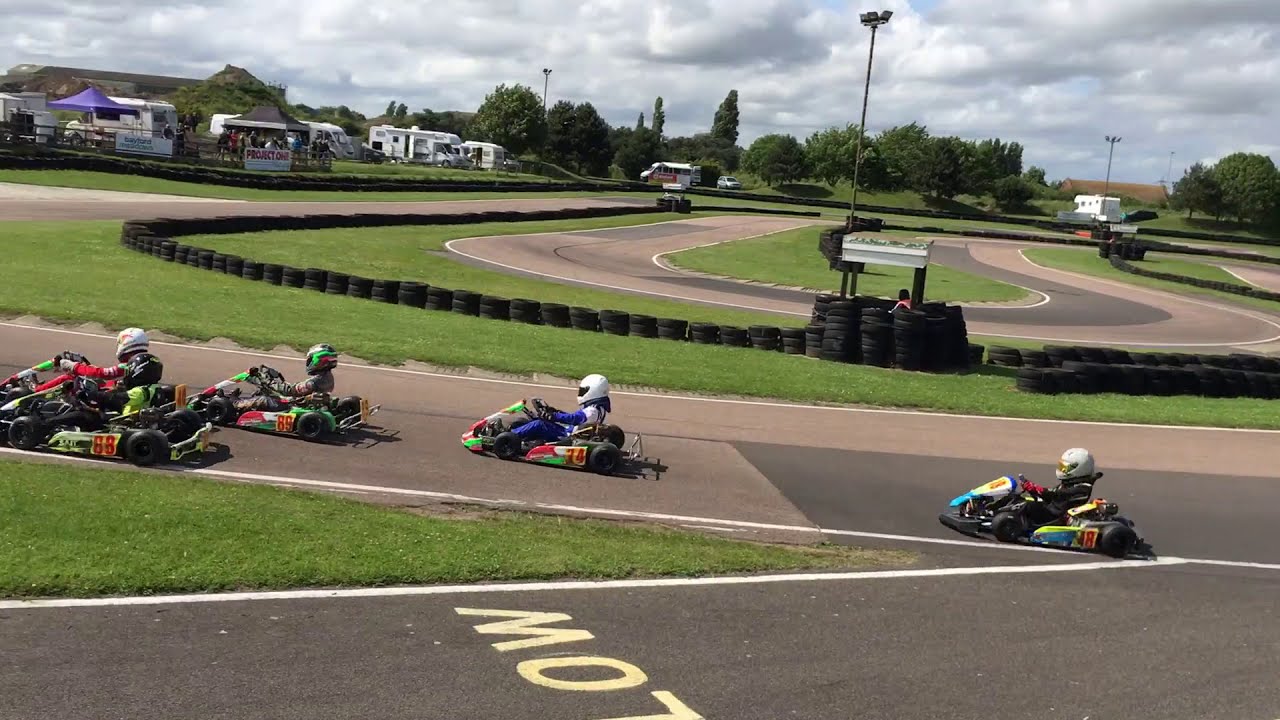In this vibrant exterior shot taken at a professional go-kart race park, several go-karts—adorned in green, yellow, red, and blue hues—whiz around an extensive track marked by looping curves and solid white lines. The track, surfaced in a pinkish-gray asphalt, is bordered by a barrier of black tires separating the racing area from surrounding grass and dirt. The racers, clad in helmets and colorful racing gear, navigate at high speed through the course. Notable details include a go-kart numbered '88' decorated in yellow, black, and green, and another marked '89' in lime green, white, and red. In the background, an outdoor event unfolds, featuring canopies, blue tents, and white RVs, along with kiosks bearing sponsor logos like "Project One." The sky above is overcast, adding a moody backdrop to the scene, while towering green trees frame the landscape, enhancing the impression of a resort setting. The word "SLOW" is partially visible on the track, hinting at the safety measures in place amidst the spirited competition.